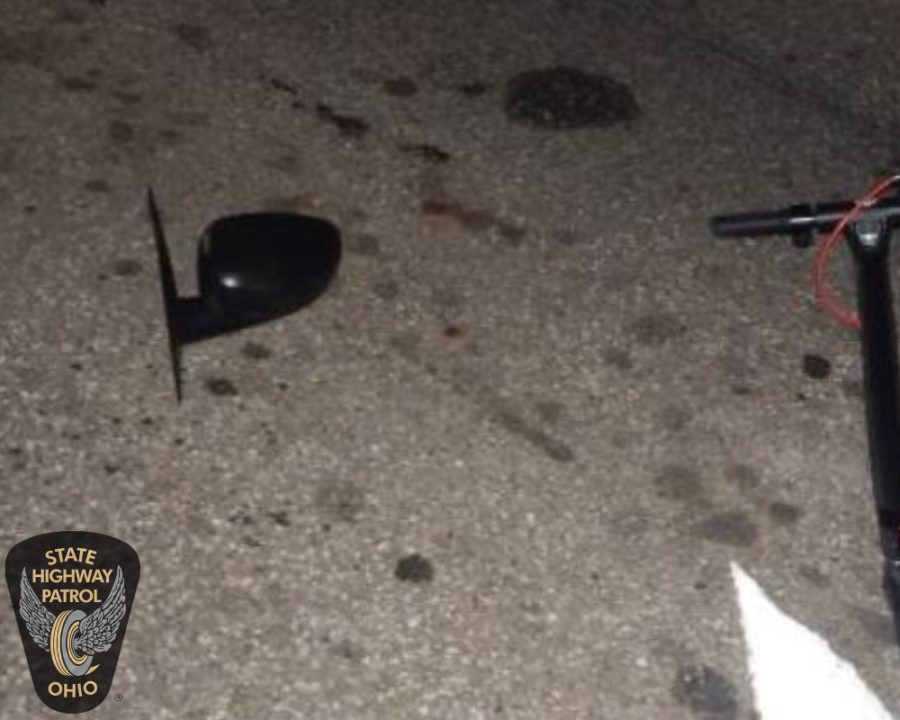The image depicts a roadside scene under investigation by the Ohio State Highway Patrol, as evidenced by the emblem and text "State Highway Patrol Ohio" in yellow lettering on a black background in the lower left corner. Prominently featured in the center is a black car side-view mirror lying on the gray, asphalt road, suggesting it may have been clipped off during an accident. Surrounding the mirror are dark spots on the ground, possibly indicating blood and oil stains. To the right side of the image, there is a device resembling handlebars, wrapped with a red cord, potentially part of a scooter or similar transportation equipment.